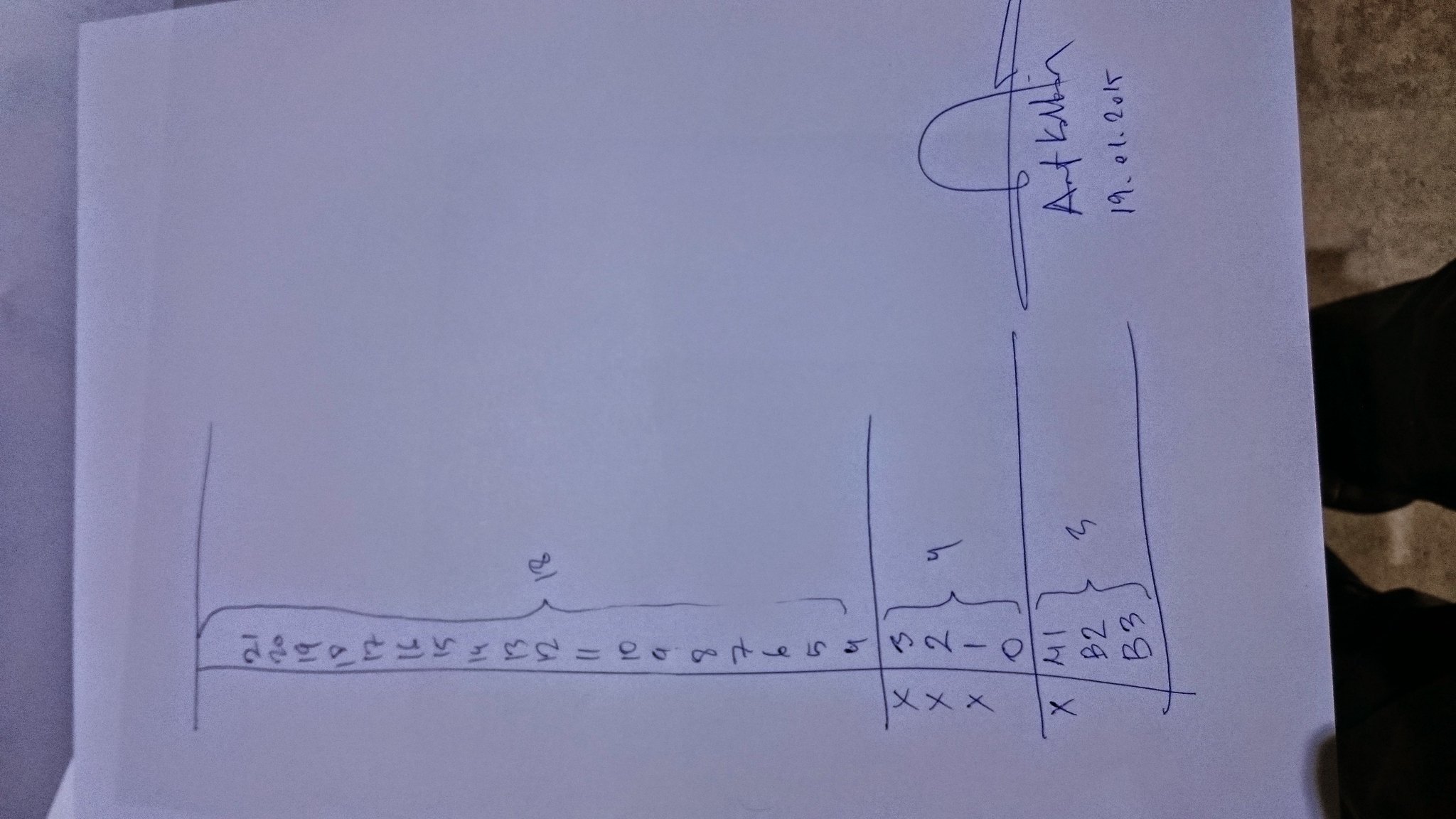This photograph features an off-white piece of paper with a drawing created using an ink pen. The drawing consists of a horizontal axis displaying a series of numbered intervals, starting at 21 and descending sequentially through 20, 19, 18, 17, 16, 15, 14, 13, 12, 11, 10, 9, 8, 7, 6, 5, 4, 3, 2, 1, down to 0. Above the number 4 is a parenthesis enclosing the number 18, and another parenthesis appears above 0 containing the number 4. To the left of this number line, there are three X's marked. 

Further below the main segment, the drawing includes a notation that reads "41B2B3," where there is an X next to "41" and a number 3 following it. The bottom segment of the paper concludes with an indecipherable signature, dated "19.01.2015".

In the photograph, the paper is being held, likely by the person taking the picture. To the right-hand side of the image, the lower legs of the individual holding the paper are visible against a tan-colored floor.